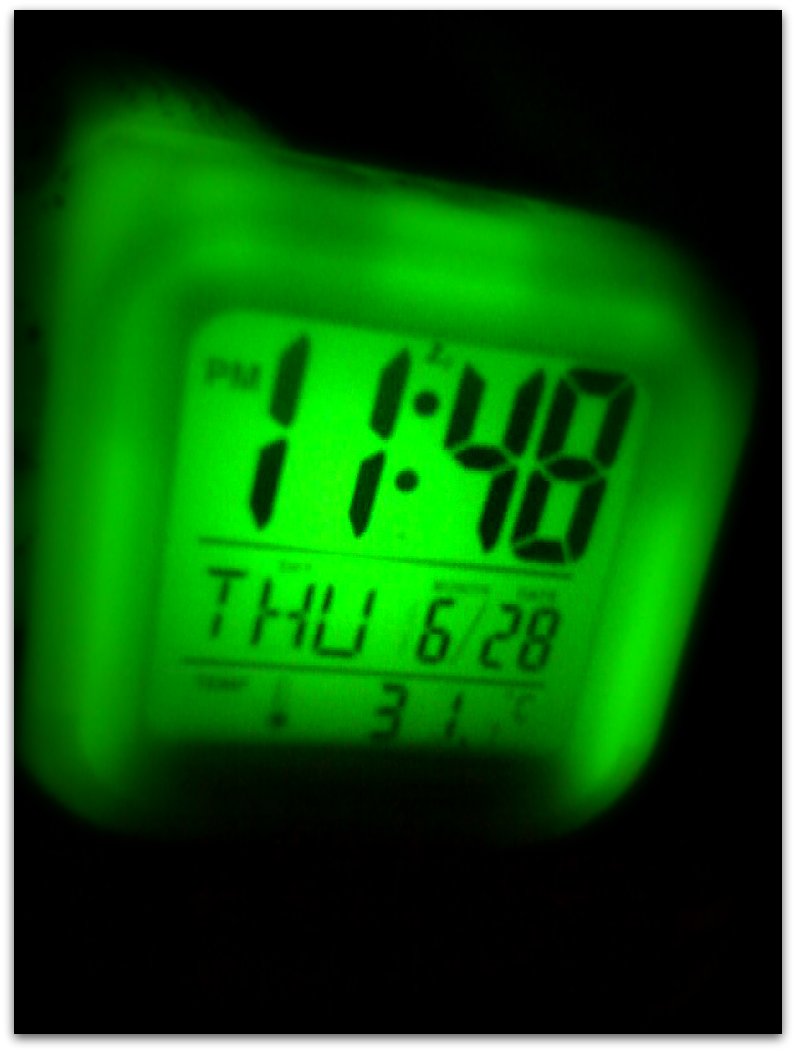The image is a close-up of a digital watch, brightly illuminated in green against a stark black background. The time displayed is 11:48 PM, prominently shown in digital black print. The day of the week, "Thursday," is also indicated in an abbreviated form as "THU." Below the time, the date is marked as "6/28," separated by a slash. Additionally, there's a temperature reading displayed with a small thermometer icon beside it, reading "31°C." The overall display is brightly lit in green, standing out vividly against the dark backdrop. The precise details suggest it could be either a digital watch or a wall-mounted thermostat.